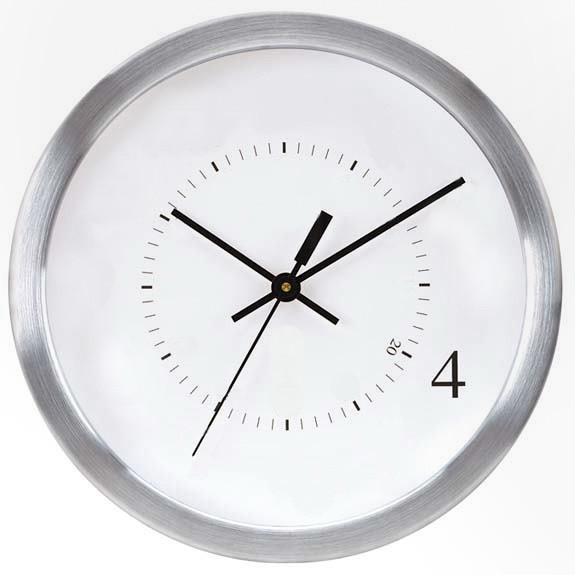This image features a circular clock set against a pristine white background. The clock boasts a brushed silver frame, roughly an inch thick, creating an elegant border. The time displayed is approximately 10:10, with black hour and minute hands, complemented by a black second hand. The clock face is minimalist, adorned with tick marks in place of numbers, except for the number 4 at its traditional position. Additionally, a smaller Arabic numeral 20 is located just to the left of the 4, potentially indicating seconds.